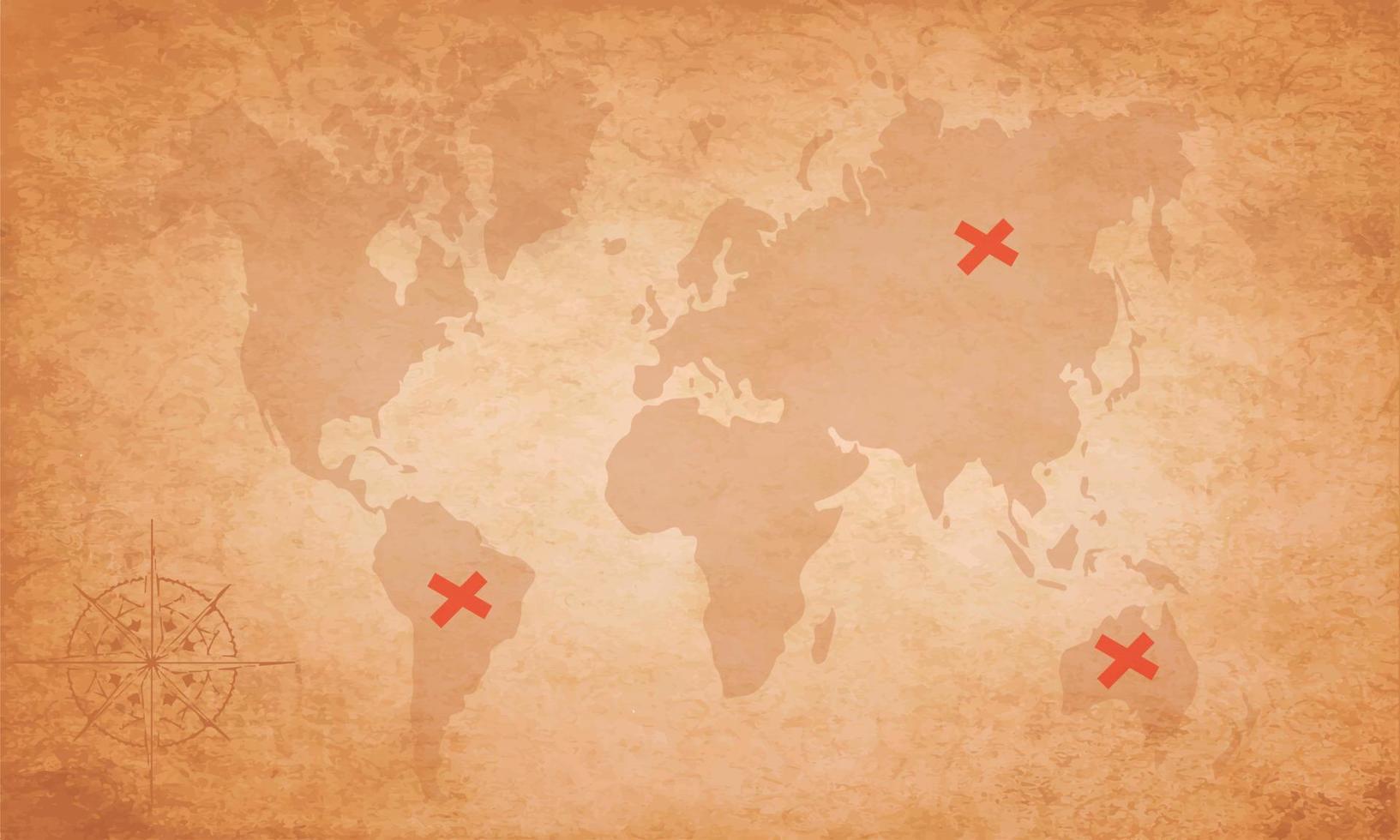This illustration depicts a weathered, antique-style world map rendered in varying shades of brown and tan, giving it the appearance of aged paper with a patina. The outlines of Earth's continents are subtly darker than the background, requiring careful scrutiny to discern their shapes. A compass symbol adorns the lower right-hand corner of the map. Distinctively, three bold red X marks are placed on specific locations: one over South America, one within northern Russia, and one over Australia. Unlike modern maps, this illustration lacks country borders, city markers, and other detailed annotations, focusing solely on the continents' rough outlines and the striking red Xs.